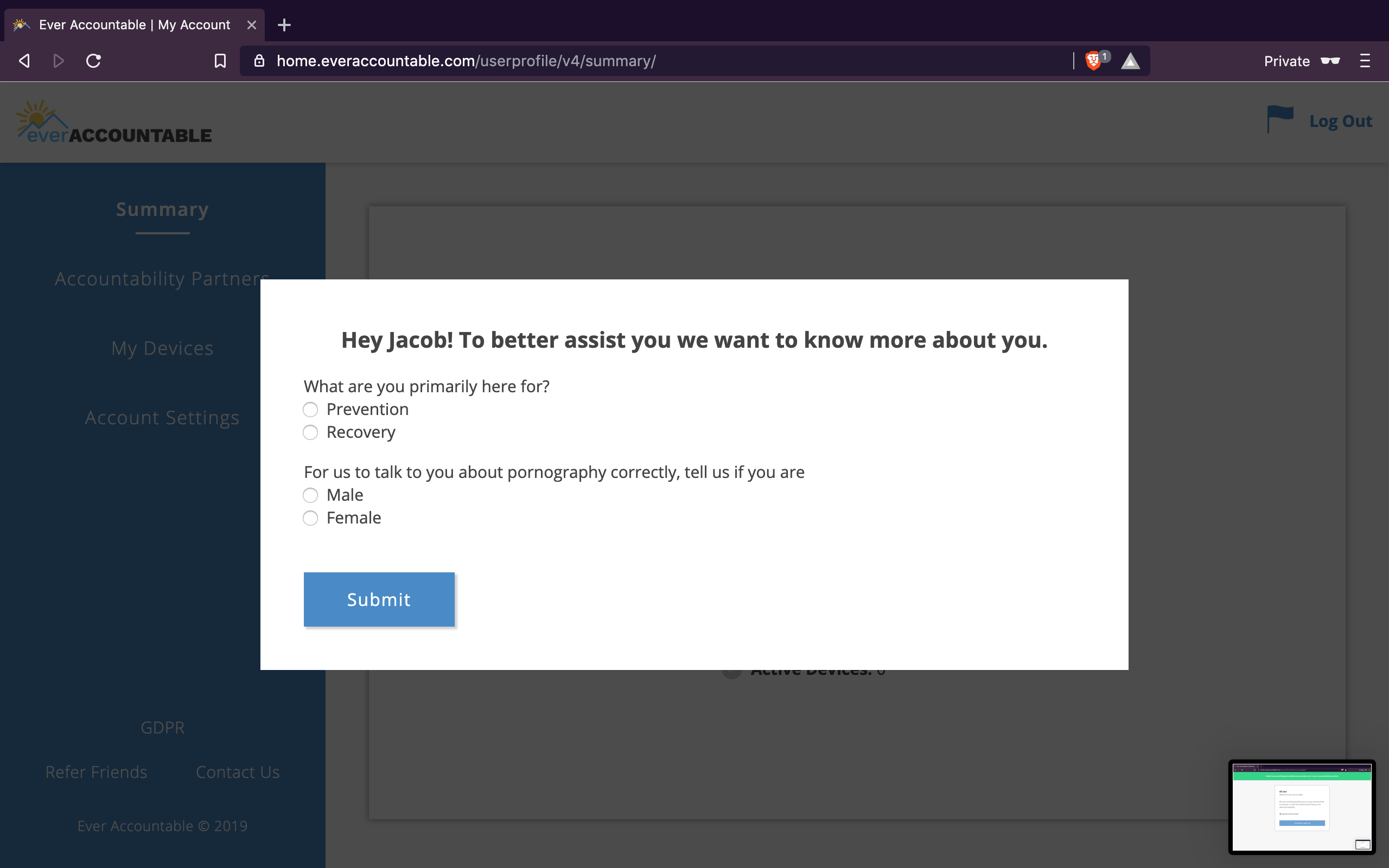The image depicts a web page from the URL home.everaccountable.com. At the center of the page, there is a prominent white pop-up menu with black text addressing a user named Jacob. The text reads: "Hey Jacob, to better assist you, we want to know more about you. What are you primarily here for?" It offers two options for selection: "prevention" and "recovery," with neither option currently selected. It continues, "For us to talk to you about more pornography, correct, tell us if you are male or female." Again, no option is selected. At the bottom left of the pop-up, there is a blue "Submit" button.

On the left side of the page, the main website navigation is visible with a blue background and white text. The menu items include: "Summary," "Accountability Partner," "My Devices," "Account Settings," "GDPR," "Refer Friends," "Contact Us," and "Ever Accountable © 2019." At the top left, the site logo is displayed, featuring the name "ever accountable," with "ever" in blue and "accountable" in black. Above the text is a blue drawing of a mountain with a yellow sun and sun rays.

The main page content, partially obscured by the pop-up, has a white background. In the bottom left corner of the main page, there is a green and white image that appears to be a screenshot.